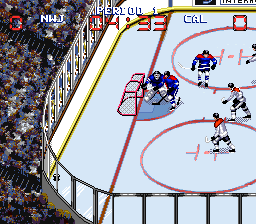This image is a low-resolution screenshot from a computer or video game depicting an ice hockey match. The clarity is poor, making finer details difficult to discern. The scene captures a small section of an ice hockey rink with six players actively engaged on the ice. A goal post is present, suggesting a focus near the net. Surrounding the rink, colorful, indistinct dots likely represent a cheering crowd. Across the top of the screenshot, there are several infographics: "Period 1," a game clock showing "04:33," and scoreboard elements displaying both teams with a score of "0-0."